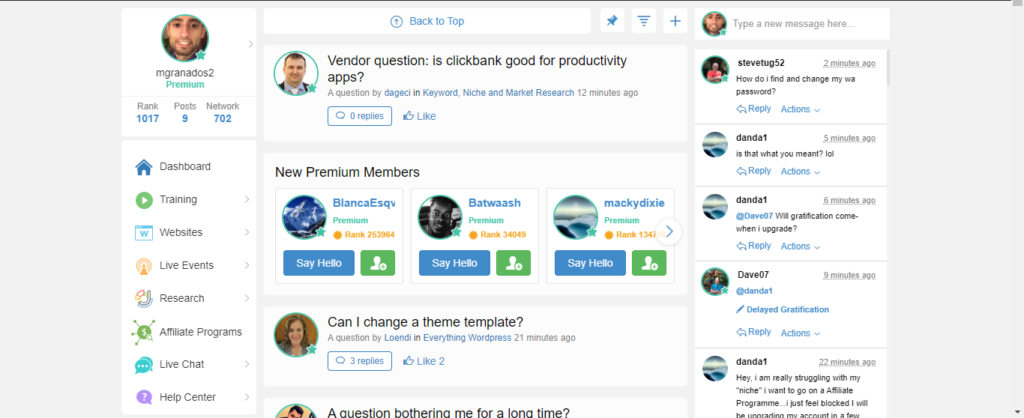This is a detailed screenshot of a website, showcasing various sections and elements. Along the right and left sides, there are grey bars, framing the main content area. The text within the screenshot is quite small, necessitating zooming to read clearly.

On the left, a user profile section features an avatar of a medium-skinned male with a beard, his username is "mygrandso2". Below his name, "Premium" is highlighted in green. He has a rank of 1017, Pulse 9, and Network 702. Directly beneath this information is a navigational list with icons for "Dashboard," "Training," "Website," "Live Events," "Research," "Affiliate Programs," "Live Chats," and "Help Centre."

In the center, a "Back to Top" button is prominent. Below it, a question about productivity apps on ClickBank is posed, accompanied by another avatar of a man in a circle. The query, made by user "Diageo," appears in the "Keyword, Niche and Market Research" category, posted 12 minutes ago with zero replies and a like option available.

Further down, there's a section introducing New Premium Members: "Blanca Esquire," indicated by a blue circle, "Batwish" represented by a black and white photo of a dark-skinned person, and "Mackie Dixie," whose picture showcases the sea and sky. Visitors are prompted to greet these new members, and a "friend" button is visible.

A subsequent query is posted by a female user "Lewindi" in the "Everything WordPress" category, asking if she can change a theme template, 21 minutes ago. Another partially visible question below hints at ongoing concerns, beginning with "A question bothering me for a long time."

On the top right, the user’s account details reappear with an option to type messages. Below this, a list of ongoing messages includes: 
- "Steve, Tug52: How do I find and change my WA password?"
- "Dan.1: Is that what you mean?"
- "Dan.1: Dave87, will gratification come when I upgrade?"
- "Dave07: Delayed gratification."
- "Dan.1: Hey, I am really struggling with my niche. I want to go and affiliate program. I just feel blocked."

The bottom portion of the text is cut off and unreadable.